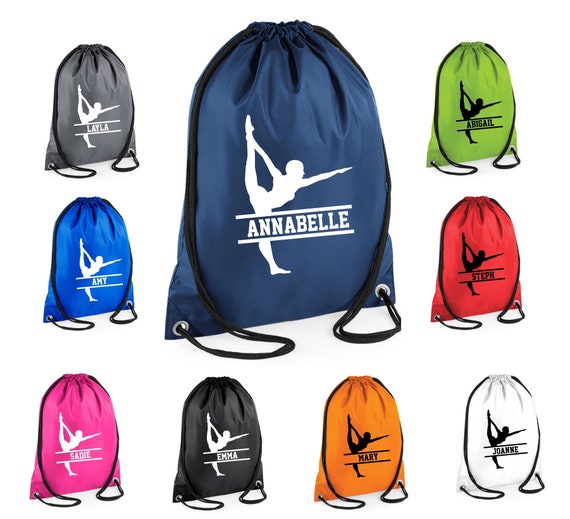This image showcases a collection of customizable drawstring backpacks, each featuring a dancing figure design. The backpacks, which come in various colors such as gray, blue, pink, orange, green, navy, white, and black, have names printed on them, including Annabelle, Joanne, Steph, Amy, Sadie, Layla, Emma, Mary, Joey, and Abigail. In the center of the photograph is a larger navy blue backpack with black drawstrings, adorned with the name "Annabelle" in white letters flanked by two horizontal lines. The dancing figure, depicted with arms extended and touching an ankle in mid-air, is consistently represented on all the bags. While the bags on the right side of the image feature the silhouette and lettering in black, others have the figures and names in white. The overall theme of the image highlights the bags' customizable nature, suitable for a product listing.